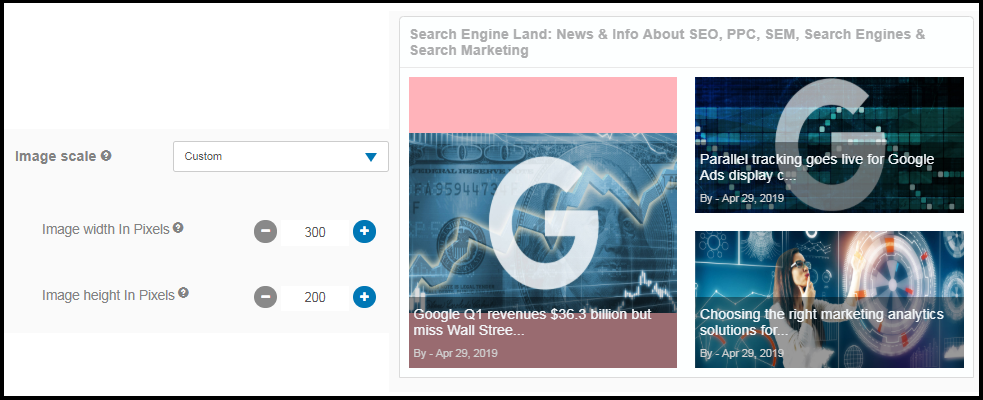Descriptive Caption:

The website interface displays a range of features for customizing the image scale and dimensions. On the left side, there is an elongated horizontal white box with the text "Image Scale" followed by a question mark, indicating help is available. Adjacent to this is a dropdown menu labeled "Custom," allowing the user to select alternative scaling options.

Below, the interface presents options to modify the image's dimensions. The "Image Width in Pixels" is currently set to 200 pixels, with blue and grey buttons for increasing or decreasing the value. Similarly, the "Image Height in Pixels" is set at 200 pixels, with corresponding buttons for modification.

Towards the top right, a text box with grey lettering reads "Search Engine Land: News and Info about SEO, PPC, SEM, Search Engines, and Search Marketing," with "Search Marketing" displayed on a new line.

Below the text box is a prominent thumbnail image featuring a white "G" for Google, overlaid with stock market lines and a faint blue watermark of a $100 bill. The accompanying caption states, "Google Q1 revenue is $36.3 billion but missed Wall Street expectations...," dated April 29, 2019. Beneath this are two additional news items: one about "Parallel Tracking Goes Live for Google Ads" and the other featuring a thoughtful woman with glasses titled "Choosing the Right Marketing Analytics Solution," both dated April 29, 2019.